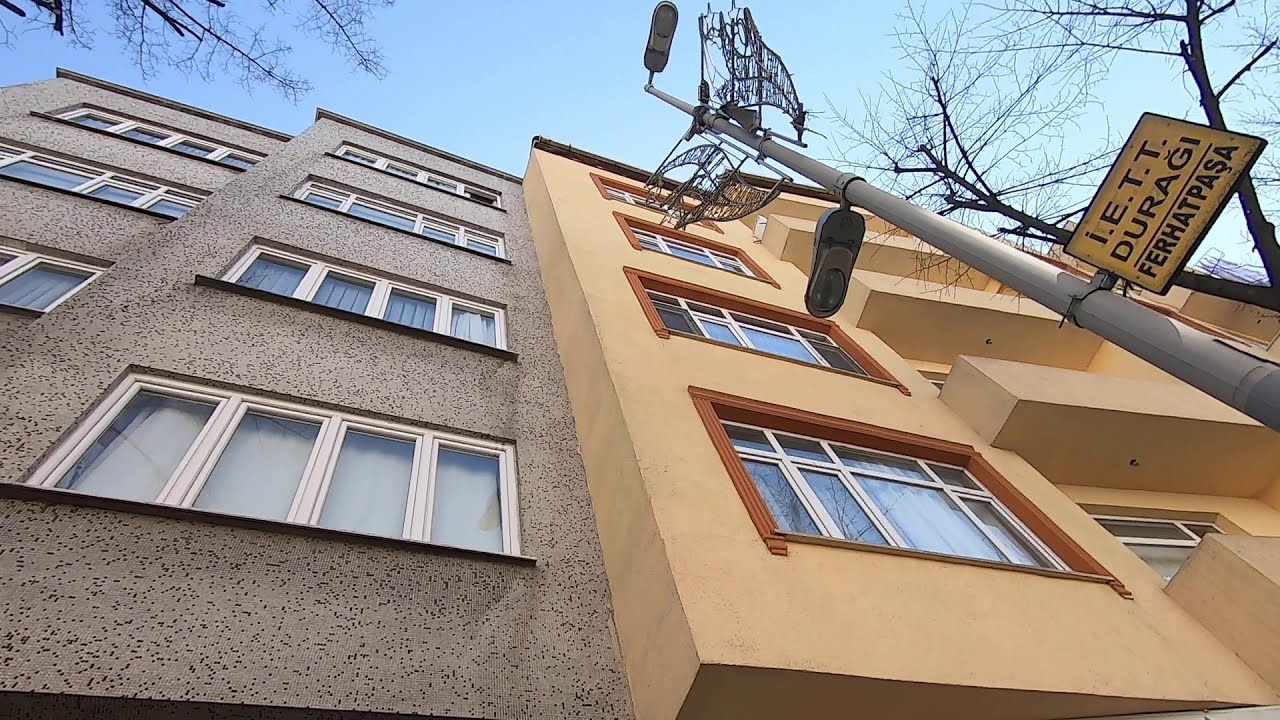The image captures a perspective from the ground looking almost straight up the side of a multi-story, stucco building. The building has two distinct color sections: the right side is a very light orange with windows framed in rust-colored panels divided into four panels each by white vertical bars, while the left side is a granite color with less prominent window frames. This side is slightly indented compared to the right. Four floors are visible, each with one set of staggered windows aligned in a pattern where the rightmost section protrudes slightly more than the left.

In the foreground, there’s a silver metal pole topped with an unlit light fixture featuring two bulbs. Attached to this pole is a yellow sign with black text reading "IETT Duraghi" with a vertical bar underneath followed by "FERHATPAŞA." Surrounding the scene are leafless trees, and in the background, a clear, perfectly blue sky completes the image. The setting appears outdoors, possibly midday, next to an apartment building. The overall color palette includes gray, black, tan, orange, white, yellow, and light blue.